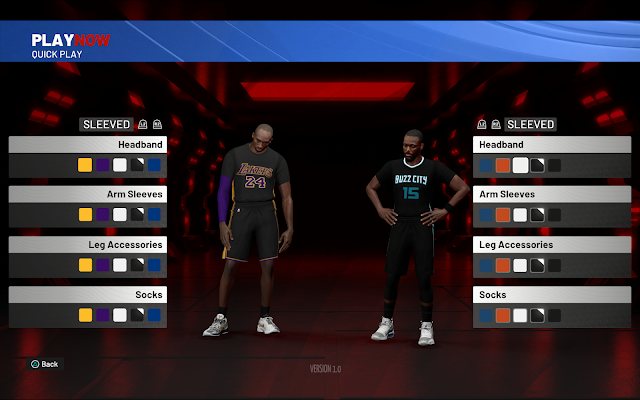This image appears to be a screenshot from an online sports game, specifically a basketball-themed title. The screen prominently displays two player characters, both of whom are Black and donning unique jerseys. The player on the left is wearing a black uniform with a white number "24" on his chest and features a distinctive purple sleeve on one arm. Conversely, the player on the right sports a jersey labeled "Buzz City 15," which has a contrasting white neckband. 

The interface allows users to customize their player avatars extensively. Options are shown for varying colors and styles of sleeves, headbands, leg accessories, and socks, enabling detailed personalization. The player on the right has chosen a color scheme incorporating black, white, and orange accessories, while the player on the left's accessories include yellow, purple, white, and black. The screen also includes options such as "Version 1," "Play Now," and "Quick Play," indicating a user-friendly menu designed for easy navigation and game initiation.